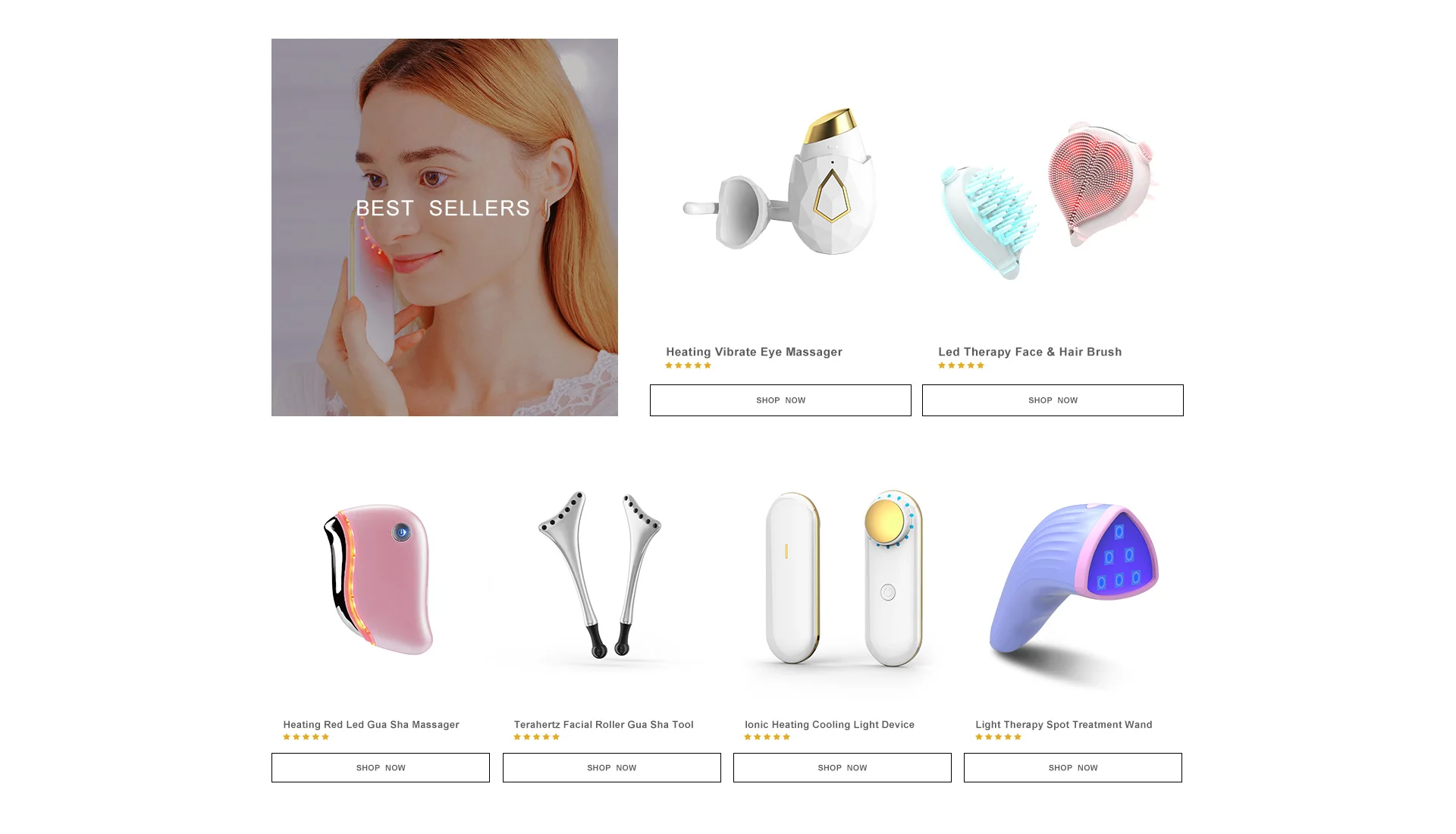The image displays an online store's "Best Sellers" section featuring a collection of six highly-rated beauty products. In the top left, a woman with bronze hair, facing left, is using a white face massage product. The central text reads "Best Sellers" in white font against a transparent background. 

1. At the top center, there is a white and gold "Heating Vibrate Eye Massager" with a 5-star rating, marked by yellow stars. Below this product is a "shop now" link.
2. The next product is an "LED Therapy Face and Hairbrush", available in white and pink or white and blue, both also boasting 5-star ratings.
3. Following this is a pink, black, and orange "Heating Red LED Washer Massager".
4. The fourth product is a silver and black "Head Facial Roller Washer Tool".
5. Next, a white, blue, and yellow "Iconic Heating Cooling Device" is displayed.
6. Finally, a purple and pink "Light Therapy Spot Treatment" completes the selection.

Each product features a "shop now" prompt beneath it. The overall background is white, making the products stand out clearly.